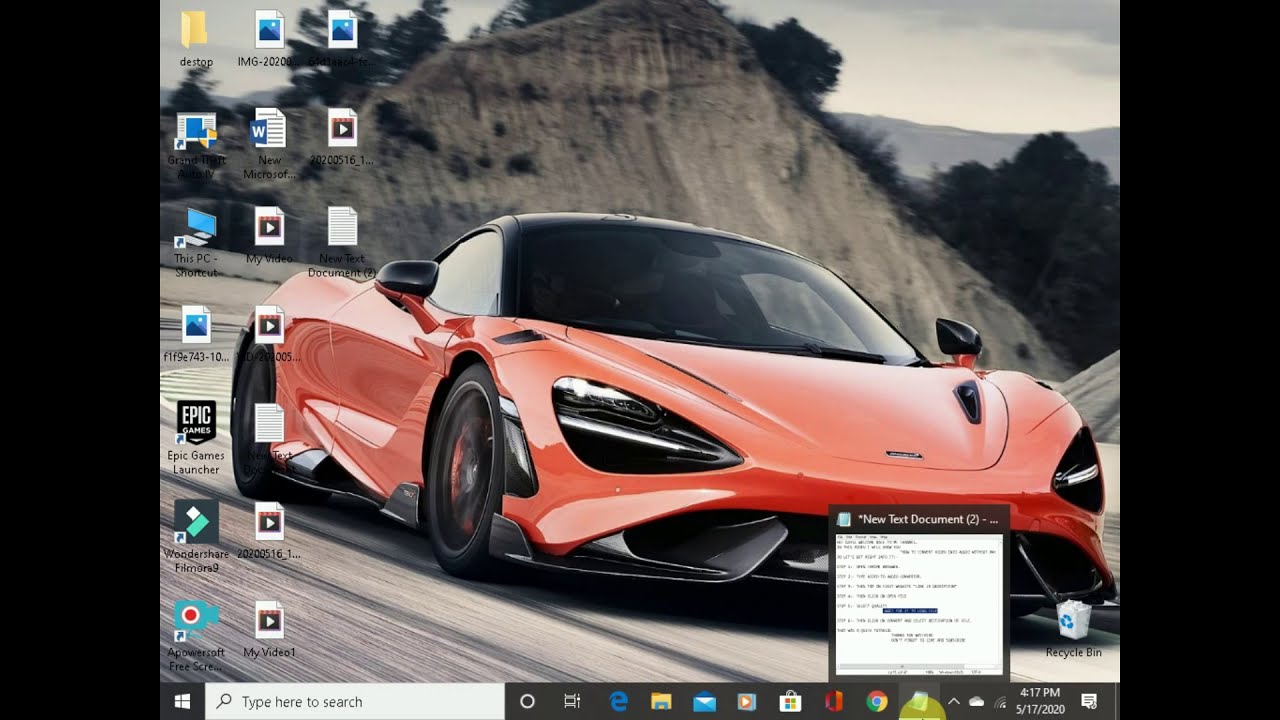The image showcases a vibrant computer desktop background featuring an orange-red sports car, possibly a Ferrari, Murcielago, or Corvette. The car, depicted in a dynamic front-angled view with shiny, natural light reflections, has distinctive black features including a bumper, tinted headlights, side mirrors, and rims. It appears to be speeding along a highway through a desert landscape with stone hills or mountains in the background. 

The computer screen, observed at 4:17 p.m. on May 17, 2020, contains several icons on the left side organized into three vertical columns. Common icons displayed include Internet Explorer, Outlook, Firefox, and Google Chrome. The taskbar at the bottom shows a menu and a pop-up covering the car's front license plate, suggesting the mouse is hovering over an icon. The recycling bin is also visible at the bottom right corner of the desktop. The color palette in the image includes shades of orange, brown, gray, green, blue, yellow, light blue, aqua, white, and black.